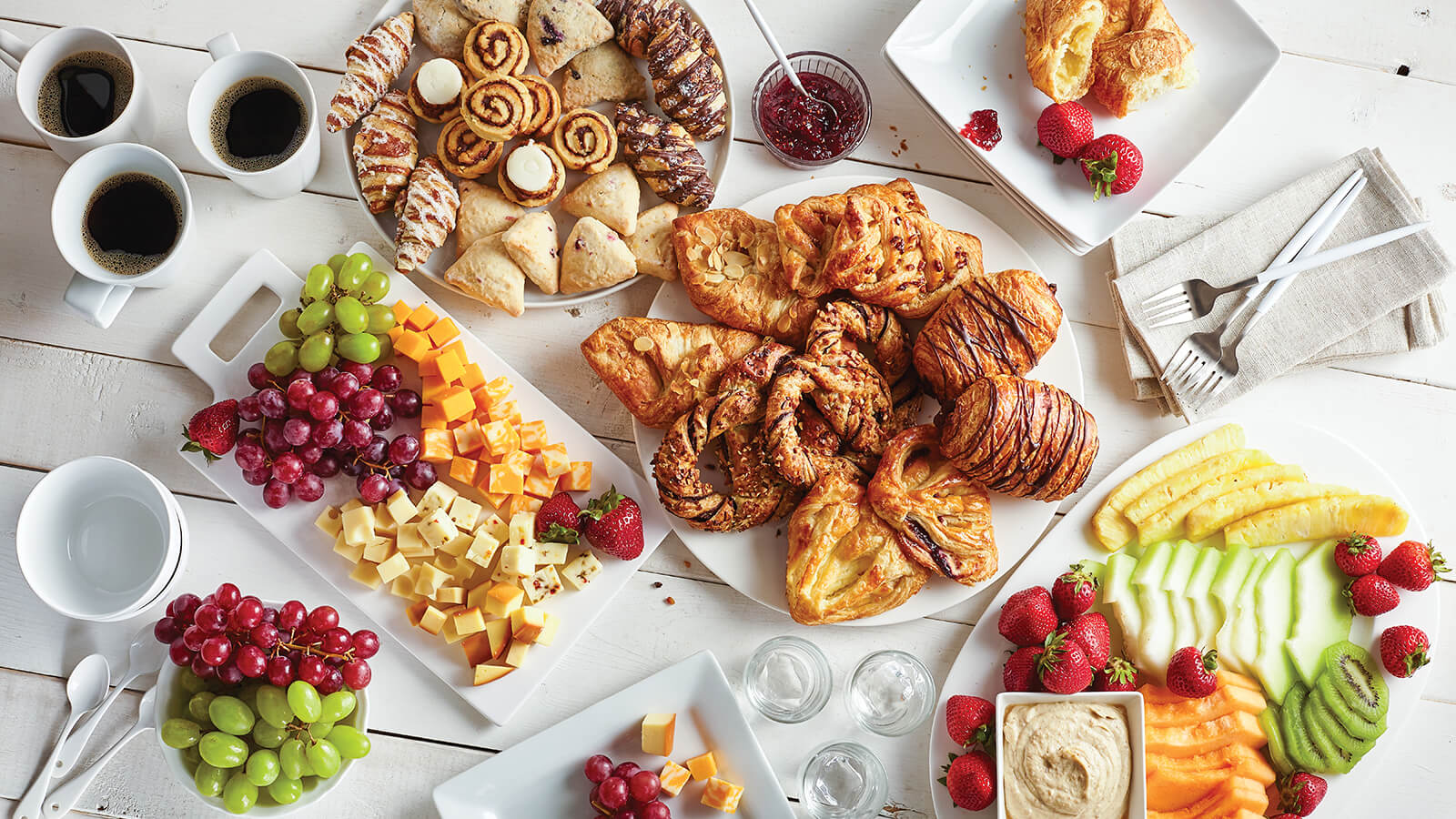The image depicts a lavish brunch spread arranged on a white wooden table. At the center, there's a platter of various flaky pastries drizzled with chocolate. To the top left, there are additional pastries, including cinnamon rolls and scones, accompanied by a bowl of mixed berry jam. Just above, there's a bowl full of red and green grapes and a cutting board with cubed pepper jack, cheddar, Colby jack, and Havarti cheeses. To the right, a large platter features an assortment of fresh fruit—kiwi slices, melon, strawberries, cantaloupe, and pineapple—alongside a bowl of dip, possibly hummus. On the lower right, another platter holds more fresh fruit, including grapes, cheese, and strawberries. Scattered throughout the table, there are empty white cups, three cups of coffee, and clear empty cups. The tableware includes white empty bowls, gray forks on gray cloth napkins, and a small dish with a white spoon filled with strawberry or raspberry jam.